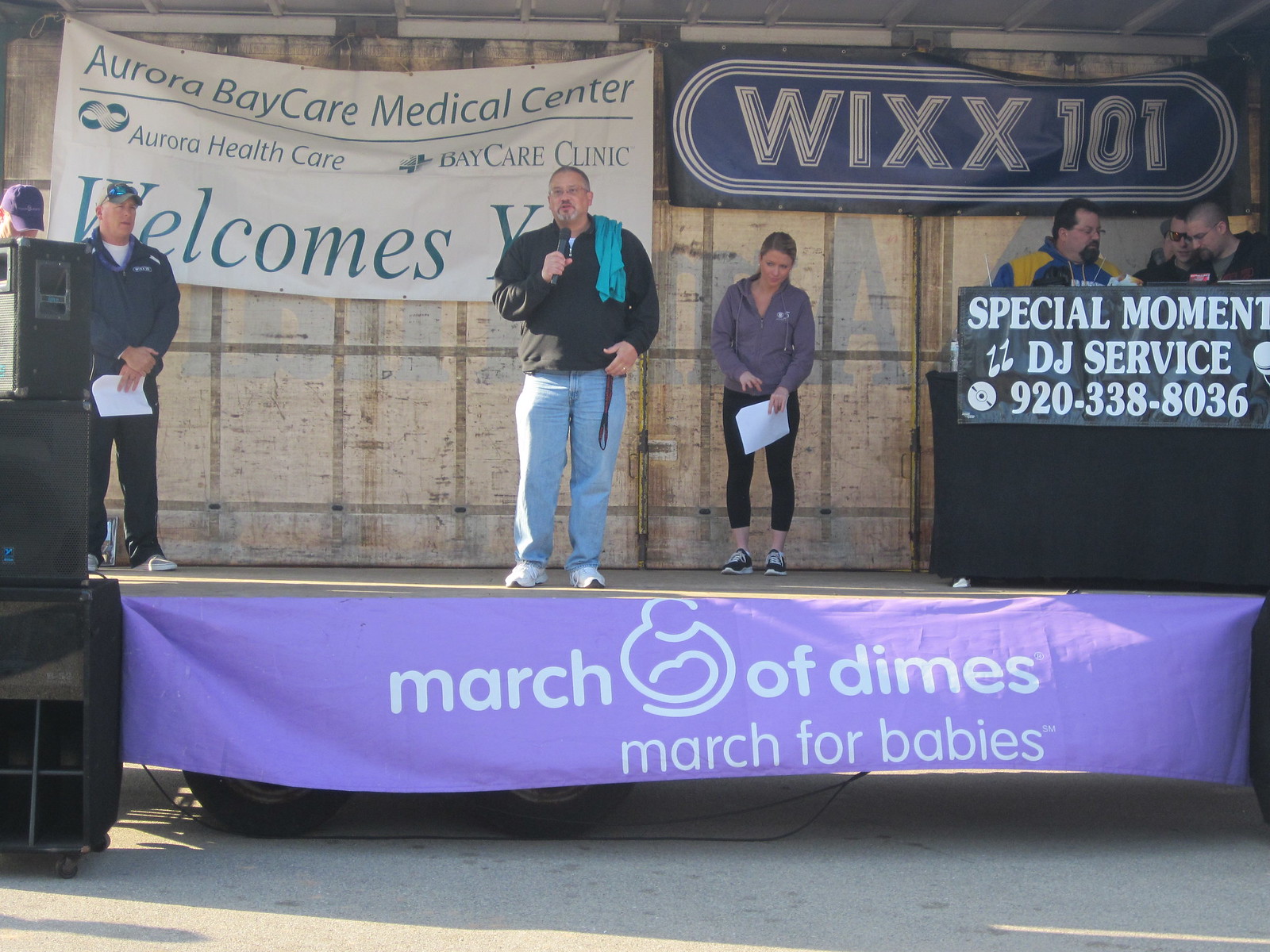The photographic outdoor image was taken during the daytime at a March of Dimes event, featuring a central stage adorned with a banner reading "March of Dimes" and "March for Babies." In the background, a sign for WIXX 101 radio station is visible alongside another banner from Aurora Health Care Medical Center welcoming attendees. At the forefront of the stage stands a man with silver hair, wearing blue jeans, white shoes, and a black jacket, holding a microphone and addressing the crowd. Draped over his shoulder is a light blue t-shirt. To his left, another man in a black jacket, white shirt, black slacks, white sneakers, and a baseball cap observes the scene. On the right, a woman dressed in black yoga pants and a purple sweatshirt holds a piece of paper while looking slightly downward. Further to the right is a desk with a sign that reads "Special Moment DJ Service, 920-338-8036," behind which sit three white men – one in a blue and yellow jacket with a mustache, goatee, and glasses, another with glasses and sparse hair, and the third also wearing glasses. The sun casts its light onto the pavement in the foreground, suggesting low-angle sunlight.